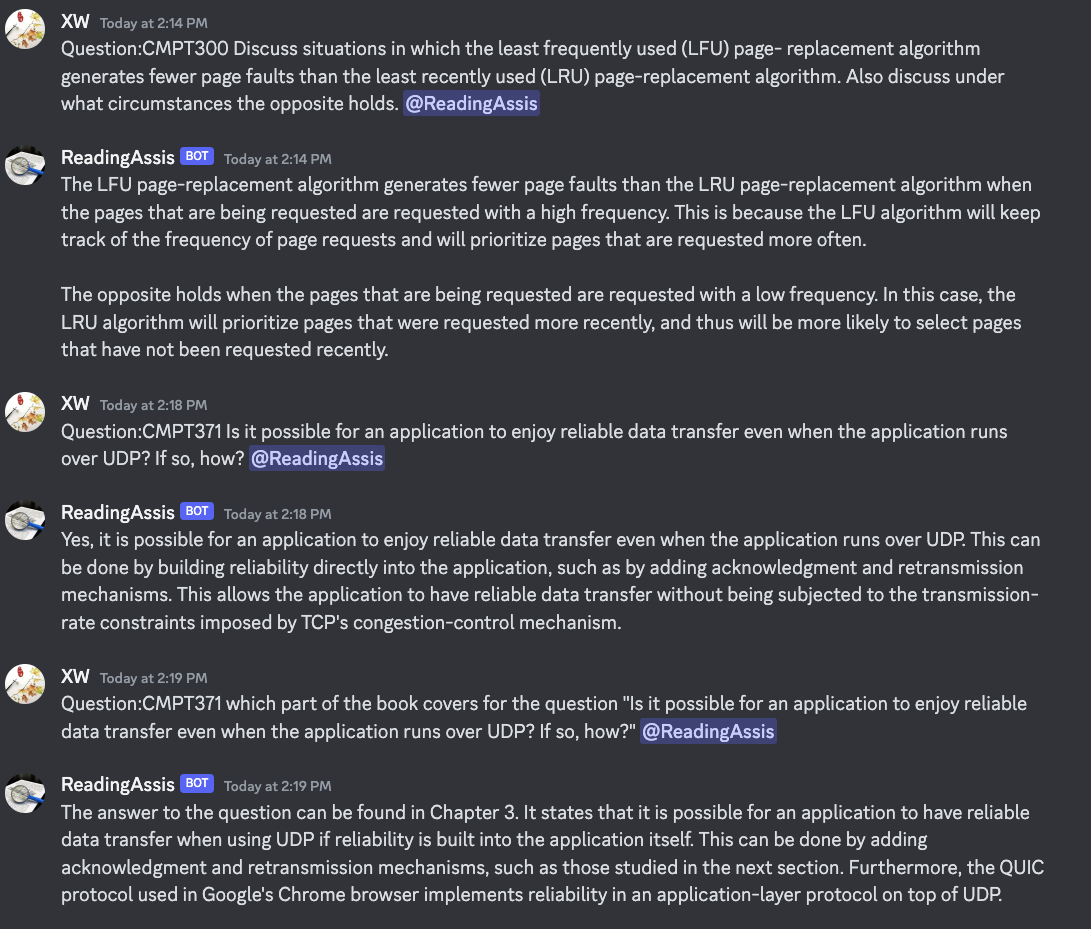A screenshot with a black background displays a message sent by a user with the initials "XW" and their profile picture included. The message, timestamped today at 2:14 PM, entailed a discussion question for CMPT-300. The user inquired about situations where the Least Frequently Used (LFU) page replacement algorithm generates fewer page faults compared to the Least Recently Used (LRU) page replacement algorithm. The message also solicited an explanation of when the reverse scenario might occur.

Highlighted within the text is a phrase, "reading assist," stylized as "ReadingAssist" with a capital 'R' and 'A' and formatted as a single word. This phrase appears in blue font. Adjacent to this, a blue rectangle that contains the word "bot" in white text is visible, indicating the participation of an automated system or bot in the conversation. 

The content of the message goes on to explain that the LFU algorithm tends to generate fewer page faults than the LRU algorithm when the pages requested have a high frequency. This is attributed to the LFU algorithm's ability to track the frequency of page requests and prioritize pages accordingly.